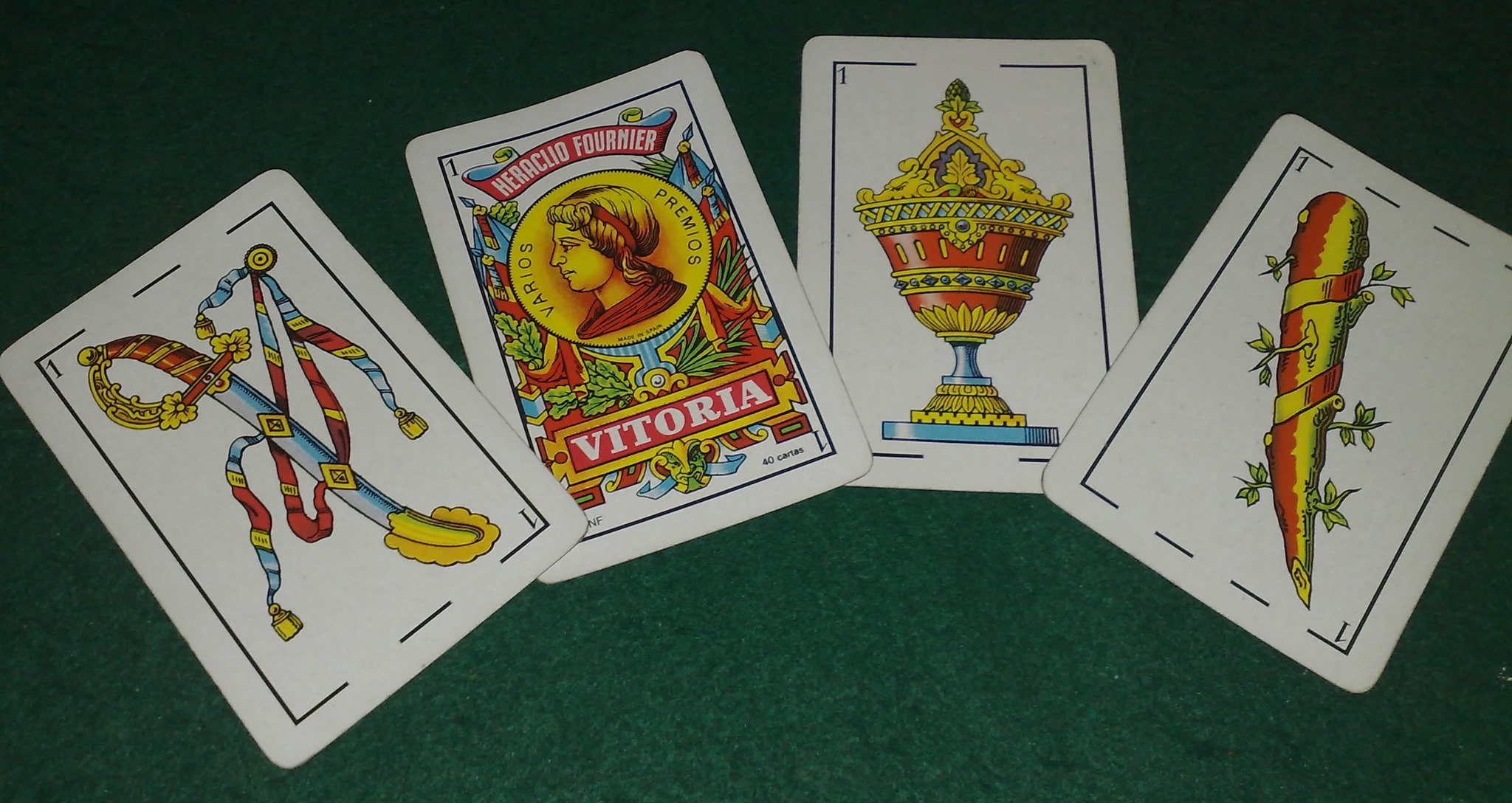The image features a quartet of intricately designed cards, each positioned atop a dark, contrasting background reminiscent of a deck of playing cards. The first card depicts an ornate sword adorned with a tie-like attachment, suggesting a ceremonial or waist-bound accessory. The second card, titled "Vitoria," showcases a figure wearing a head wrap and a vibrant red robe, set against a lush, decorative backdrop of green leaves and palms. The third card features a luxurious urn embellished with an array of jewels, predominantly in red, gold, and blue hues. The final card illustrates a peculiar root or carrot-like figure, colored in red and yellow, with green leaves sprouting from it. Each card is highly detailed and contributes to the overall mysterious and lavish feeling of the composition.